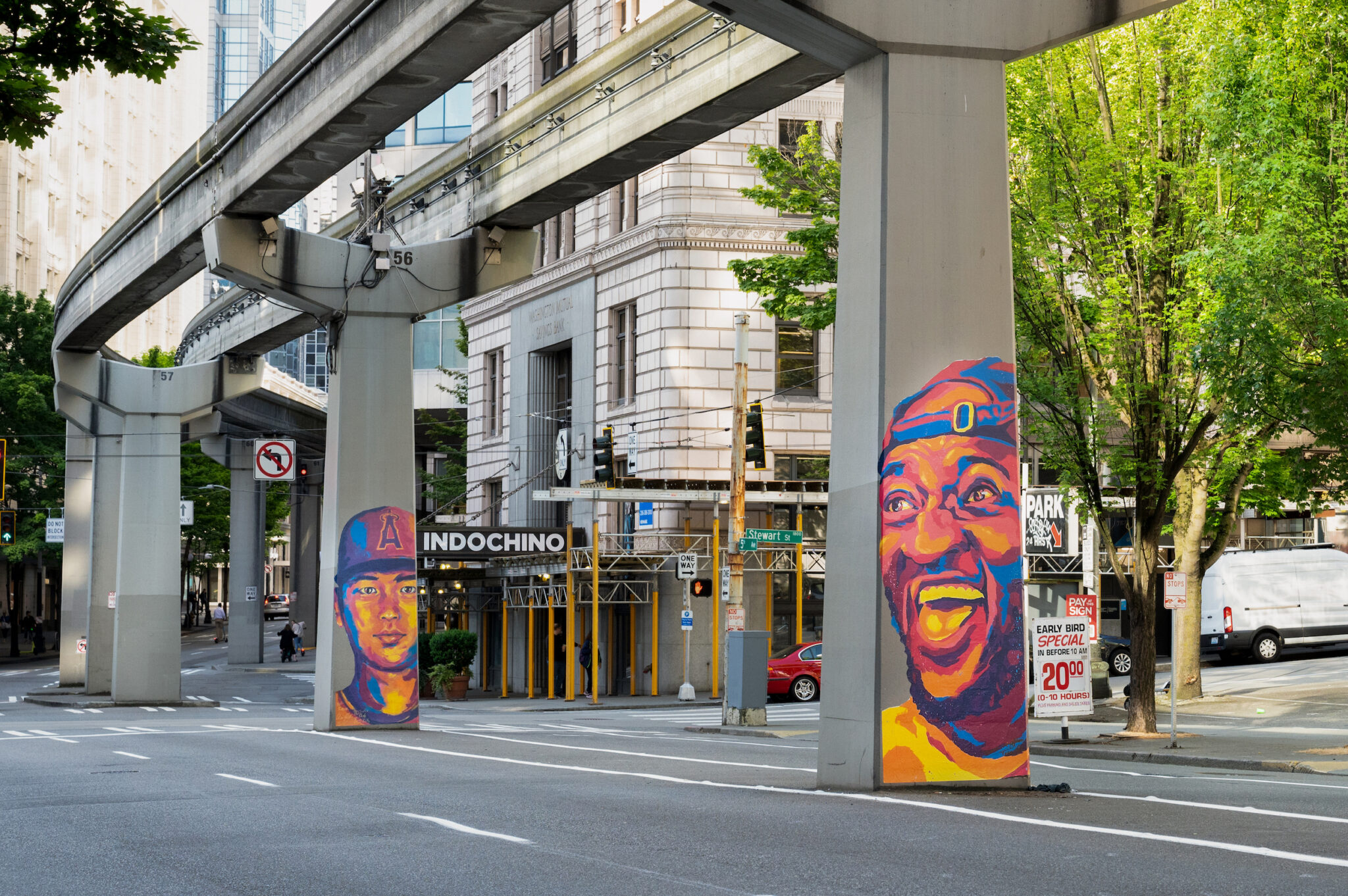In this urban street scene, the central feature is an elevated train line supported by multiple gray concrete pillars, each adorned with professional-looking graffiti. The closest pillar has a mural of a smiling person wearing a backward cap, while another nearby features a person with a hat bearing an "A," not smiling. Below the train line is a light gray asphalt road with clear white dotted lines separating the lanes and solid white lines designating the road's edges. This road curves slightly up and to the left, then back to the right in the distance. Along both sides of the street, multi-story buildings, some nearly skyscraper height, rise with varied architectural designs, including stone facades and numerous windows. 

Towards the right side of the image, a white commercial van is parked, and further along the street, a billboard and large trees punctuate the urban landscape. Additional details include traffic lights, road signs like "do not block," and various signboards, such as "early bird special," "Indochino," and "Ski World." The street also features pavements and footpaths where people can be seen walking or cycling. There's a notable corner building with scaffolding set up for ongoing work, and in front of it, a parked car adds to the bustling city environment.